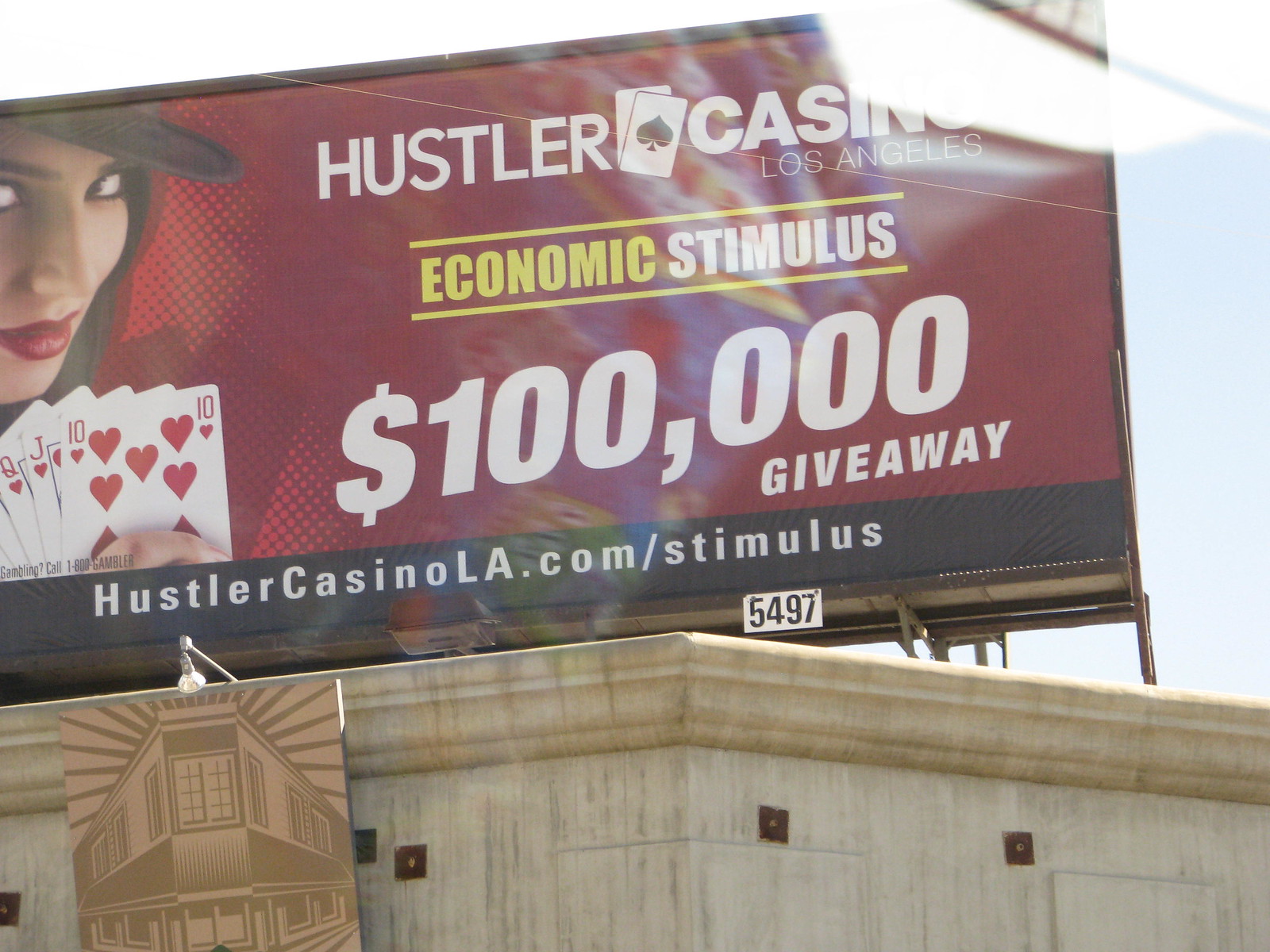In this outdoor daytime photograph, captured through a car window, the main subject is a large rectangular billboard prominently mounted atop a somewhat weathered sandstone structure. This stone platform, which might be a building or purely a base for advertisements, has a slightly dirty appearance, suggesting it could use a cleaning. On top of the stone base hangs a wooden board with a lamp, likely intended to illuminate the billboard at night. The billboard itself, slightly tilted to the left, advertises Hustler Casino in Los Angeles and features a $100,000 economic stimulus giveaway.

On the visible left side of the billboard, there is a striking image of a young, fair-skinned woman with captivating eyes and very pink lips. She wears a hat adorned with a ribbon falling over her forehead and in her left hand, she holds up a fan of playing cards, specifically the Queen, Jack, and Ten of Hearts. To the right of her image, the text "Hustler Casino" is prominently displayed in white capital letters with "Los Angeles" beneath it. Below this, the words "economic stimulus" are presented, with "economic" in yellow and "stimulus" in white, both in capital letters. Further down, "$100,000 giveaway" is written in white, and at the very bottom, a black banner reads "HustlerCasinoLA.com/stimulus," also in white capital letters. Additionally, a small white rectangle on the billboard platform itself displays the number "5497."

In the foreground, part of a concrete building with ornate trim can be seen, along with a faint reflection of the photographer wearing a multicolored blue shirt, adding a subtle, personalized touch to the image.